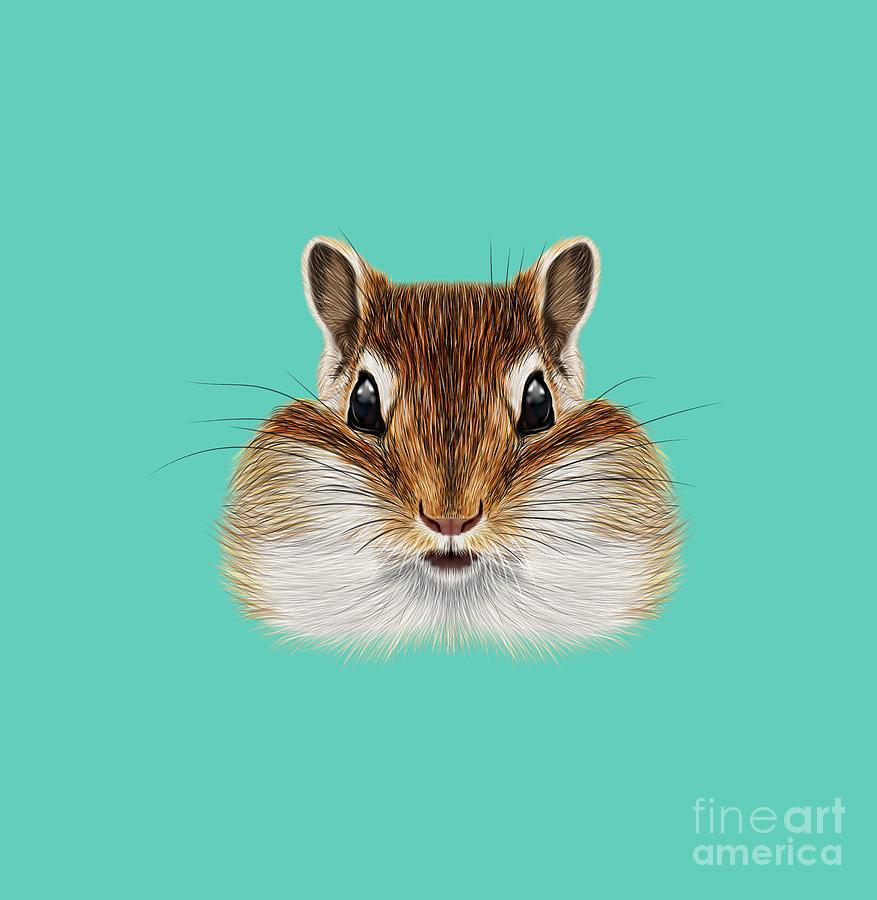This detailed and colorful graphic image features a hand-drawn squirrel or chipmunk, set against a soothing teal background. Centered is the animal’s face, exuding charm with its large, puffy cheeks and glossy black eyes. The creature, depicted in various shades of brown and white, has prominent, feathered white fur around its mouth, which appears to be slightly open. Noteworthy are its tall, alert ears and dark pink nose, complemented by black whiskers extending from its face. In the bottom right-hand corner, the phrase "Fine Art America" is printed in white, lowercase letters, with "Art America" appearing bolder than "fine," indicating a distinct printing style. This meticulous artwork beautifully captures the enchanting details of the squirrel's or chipmunk's expressive features.